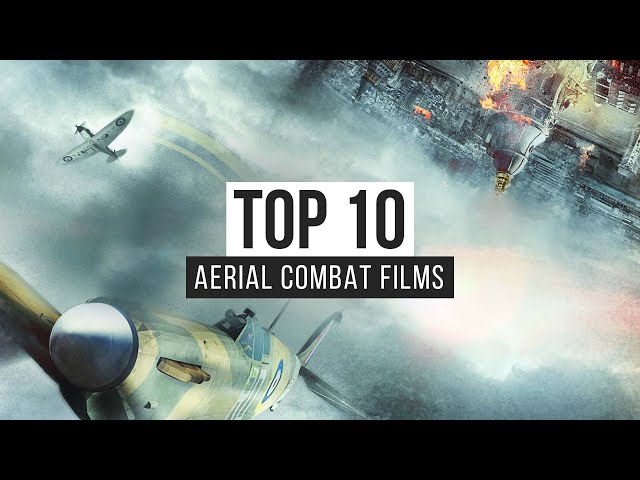The image in question appears to be a movie poster or possibly a pause screen from a video showcasing the "Top 10 Aerial Combat Films." Dominated by a sepia or muted color palette, the scene captures the essence of old war planes from bygone eras, potentially from the 1950s, 60s, or even earlier. The central focus is a World War II-era fighter jet, featuring a spinning, barely visible front propeller, located at the bottom left corner of the poster. This fighter jet is depicted flying toward the viewer and slightly to the left, armed with target symbols marked by red, white, and blue concentric circles on its body.

Towards the upper left, a second fighter jet, smaller in size but of similar design with a chrome nose cone, flies upward and away from the viewer, its own propeller discernible. This plane is showcased from behind, ascending into a sky filled with light gray and blue shades scattered with white clouds.

Adding to the dramatic atmosphere, the upper right-hand corner displays a bombed-out, cathedral-like building engulfed in flames and smoke, reinforcing the wartime theme. The structures around it are also visibly damaged and on fire. The combination of fire, cloudy skies, and misty background creates a chaotic and intense environment typical of aerial combat scenarios.

Across the middle of the poster, a white rectangle contains bold black texts: "Top 10" at the top and "Aerial Combat Films" below, encapsulating the theme of the poster. The composition, with its CG-rendered war planes and dramatic backdrop, embodies the spirit and thrill of historic aerial warfare.